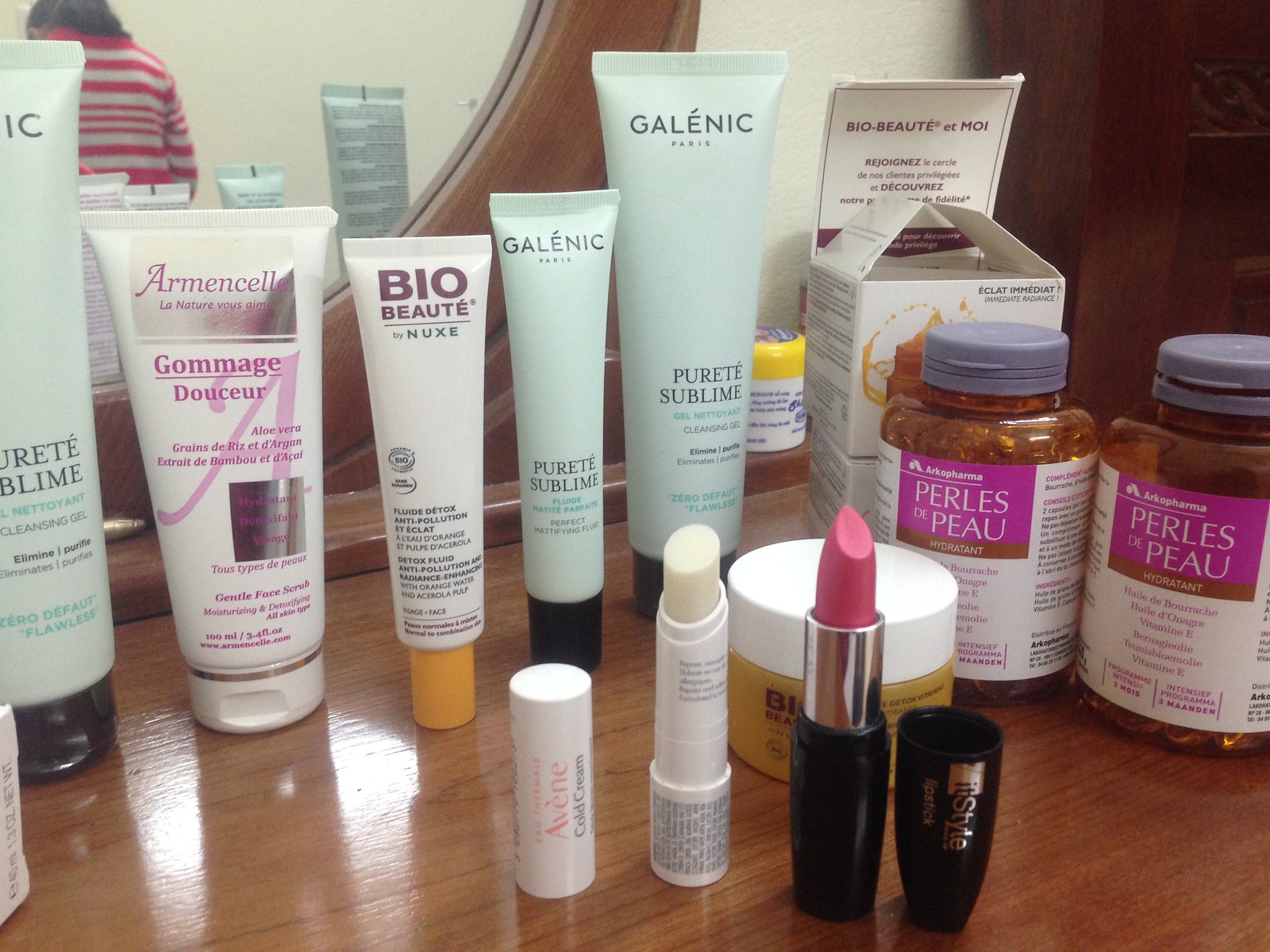This image showcases an assortment of feminine beauty and wellness products arranged neatly. In the front of the picture, there is a pink lip gloss in a sleek black container labeled "It Style," with its cap off and the lip gloss twisted up to reveal the vibrant color. Adjacent to the lip gloss is a white chapstick in a twist-up tube called "Aveen Cold Cream," intended for soothing chapped lips, especially during cold weather.

Behind these items are two transparent bottles of supplements named "Pearls de Peau," labeled as hydrating pills. The bottle on the left is full, while the bottle on the right appears partially used, revealing the visible pills inside. 

Further back, there is a white box labeled "Bio Butte et Moi Eclat Media." To its left, a blue bottle of cleansing gel stands prominently, accompanied by a mini bottle beside it, likely containing matching cleansing oil or lotion. A white tube labeled "Bio Butte" is next to them, and further left is another product named "Gommage D'Aussure Aloe Vera," indicative of an aloe vera-based exfoliating scrub. Finally, another cleansing gel bottle rounds out the extensive selection of beauty and skincare items.